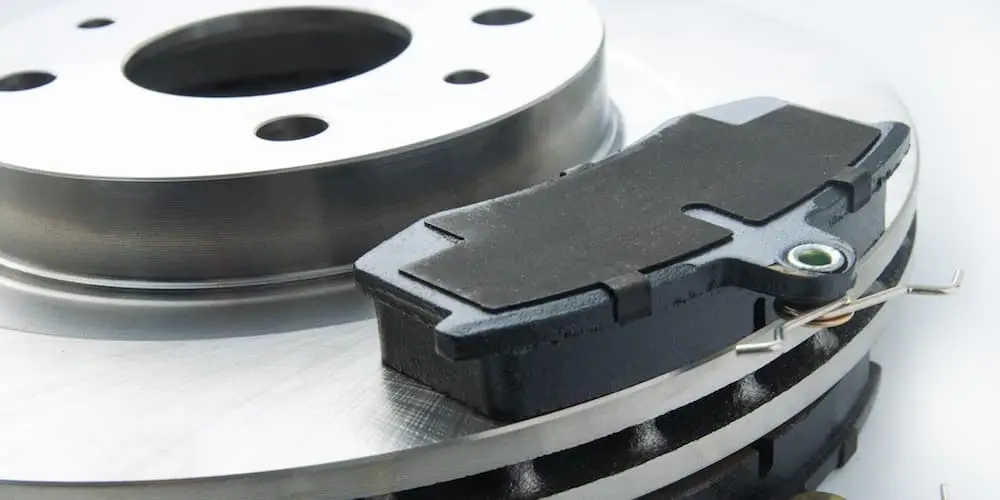This photograph depicts a close-up view of a car's brake system. Dominating the image is a silver metal brake drum with a raised platform featuring multiple holes, likely for attachment to the tire posts. On top of the drum sits a bluish-gray brake caliper accented with a solid black plate and equipped with a cotter pin-style connector. The chrome cylinder on the left side of the image has one large circle and several smaller circles, possibly indicating attachment points. The background is a plain white, emphasizing the intricate details of the brake equipment, including the dual-sided placement of the brake pads.